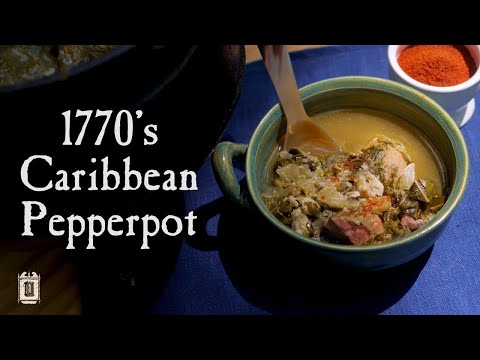The image is a YouTube video thumbnail from the channel Townsend's, which focuses on 18th-century reenactments, particularly the lifestyle, activities, and foods of the 1700s. The scene is set on a blue tablecloth, displaying a variety of culinary items. Central to the image is a greenish bowl with a handle, filled with a stew featuring pieces of beef, greens, and vegetables in a yellowish-green broth. A large wooden spoon is dipping into the stew. Nearby, there is a crock-style blue bowl and a small cup containing a deep red spice. The thumbnail is bordered by a solid black banner at both the top and bottom, and to the left of the bowl, white text reads "1770s Caribbean Pepper Pot." The image is well-lit, making the details of the dish visually appealing and perfect for a historical cooking video.